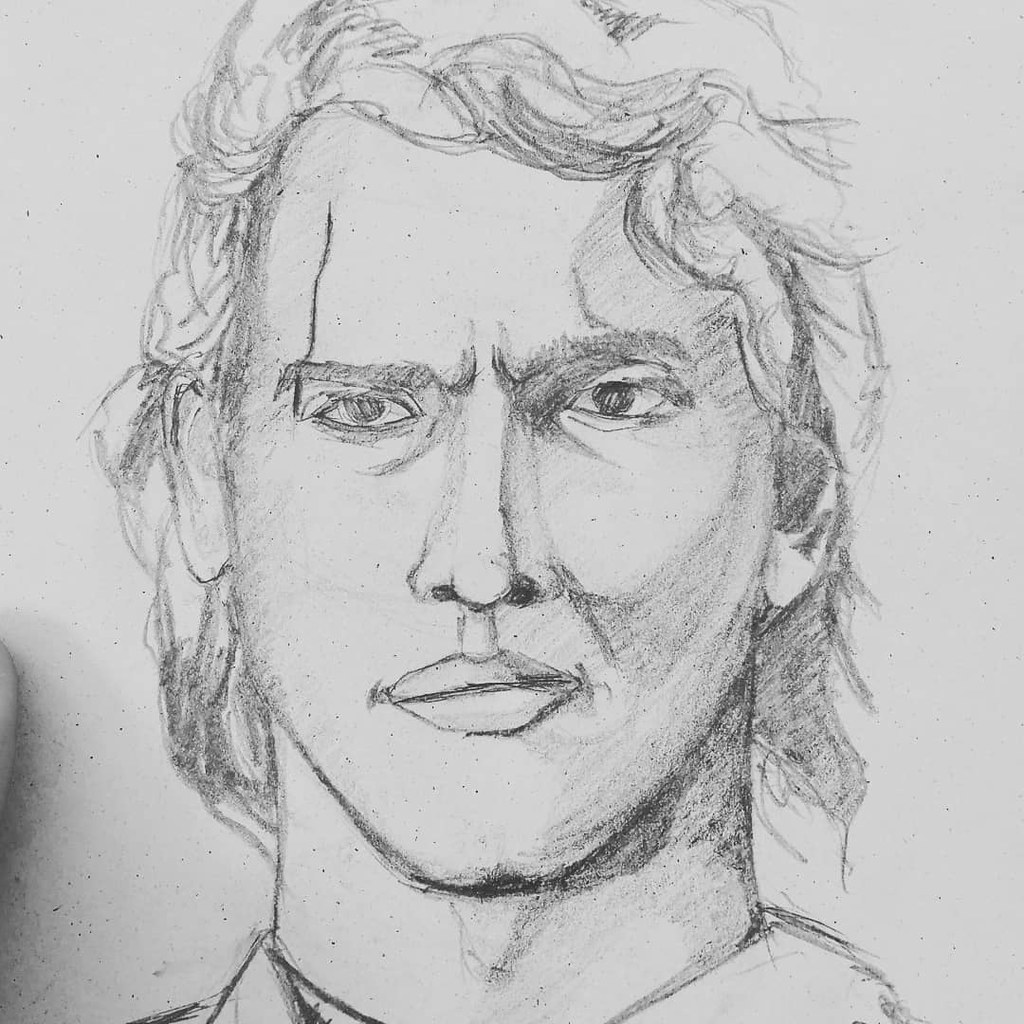This detailed black-and-white sketch, presumably created with pencil, depicts a male figure with meticulous attention to facial features and texture. The man has wavy, somewhat fluffy hair that reaches below his ears and falls slightly over the left side of his forehead. His eyebrows are clearly defined, and the artist has intensely shaded his eyes, giving them a deep, expressive look. Notably, a line runs from just below his hairline down the right side of his forehead and over his eyebrow, extending to the outer corner of his eye, possibly indicating a scar. The sketch also includes careful renderings of his nose and lips. The neck and the partial collar of a shirt are visible, suggesting he is wearing a collared garment. The entire drawing is executed in dark gray or black pencil, adding to its depth and realism. Additionally, a faint outline of what appears to be part of a finger is discernible on the far left of the image.